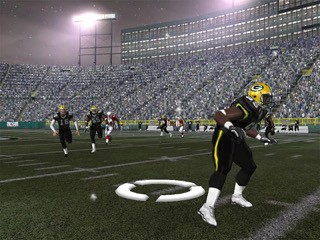The image depicts a virtual rendering of a nighttime American football game inside a stadium. The football field is marked with white lines and numbered yard markers, with a prominent 'zero' visible. The players on the field are clad in the distinctive yellow and green uniforms of the Green Bay Packers, characterized by their yellow helmets emblazoned with a white 'G' circled in green. The Packers' players also sport white socks and shoes.

Opposing the Packers, the other team is dressed primarily in white, with hints of orange or possibly another dark color on their uniforms, though the exact details are unclear. The stands are filled with crowds of spectators, suggesting a full-circle audience around the entire stadium. Visible are the luxurious boxes and suites where fans can watch the game in comfort, illuminated by the bright stadium lights mounted on dark stanchions. The atmosphere is lively and immersive, capturing the essence of an intense NFL game, albeit within the confines of a video game simulation.